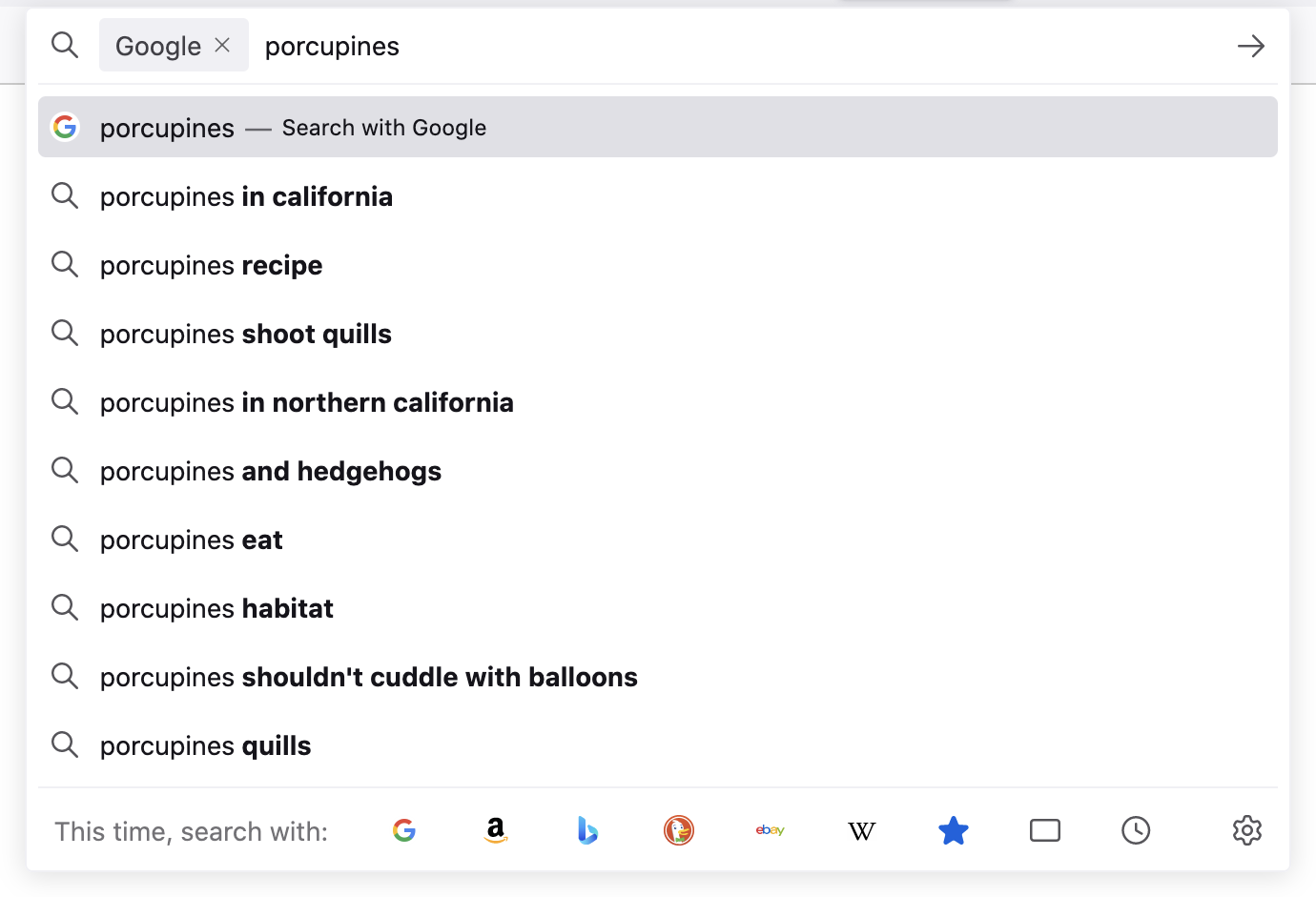A detailed screenshot of a Google search for "porcupines," showing the Google search bar at the top center of the image. The background is predominantly white with black text and light blue highlighting the first suggested search result. Beneath the search bar, there are several auto-suggested search options that include: "porcupines in California," "porcupines recipe," "porcupines shoot quills," "porcupines in Northern California," "porcupines and hedgehogs," "porcupines eat," "porcupines habitat," "porcupines shouldn't cuddle with balloons," and "porcupines quills." Below these suggestions, the image features a section titled "Search with," listing different platforms to search through, such as Google, Amazon, Bing, an unidentified icon, eBay, Wikipedia, and a starred computer icon. The interface prominently displays Google's familiar design elements, making the screenshot instantly recognizable.